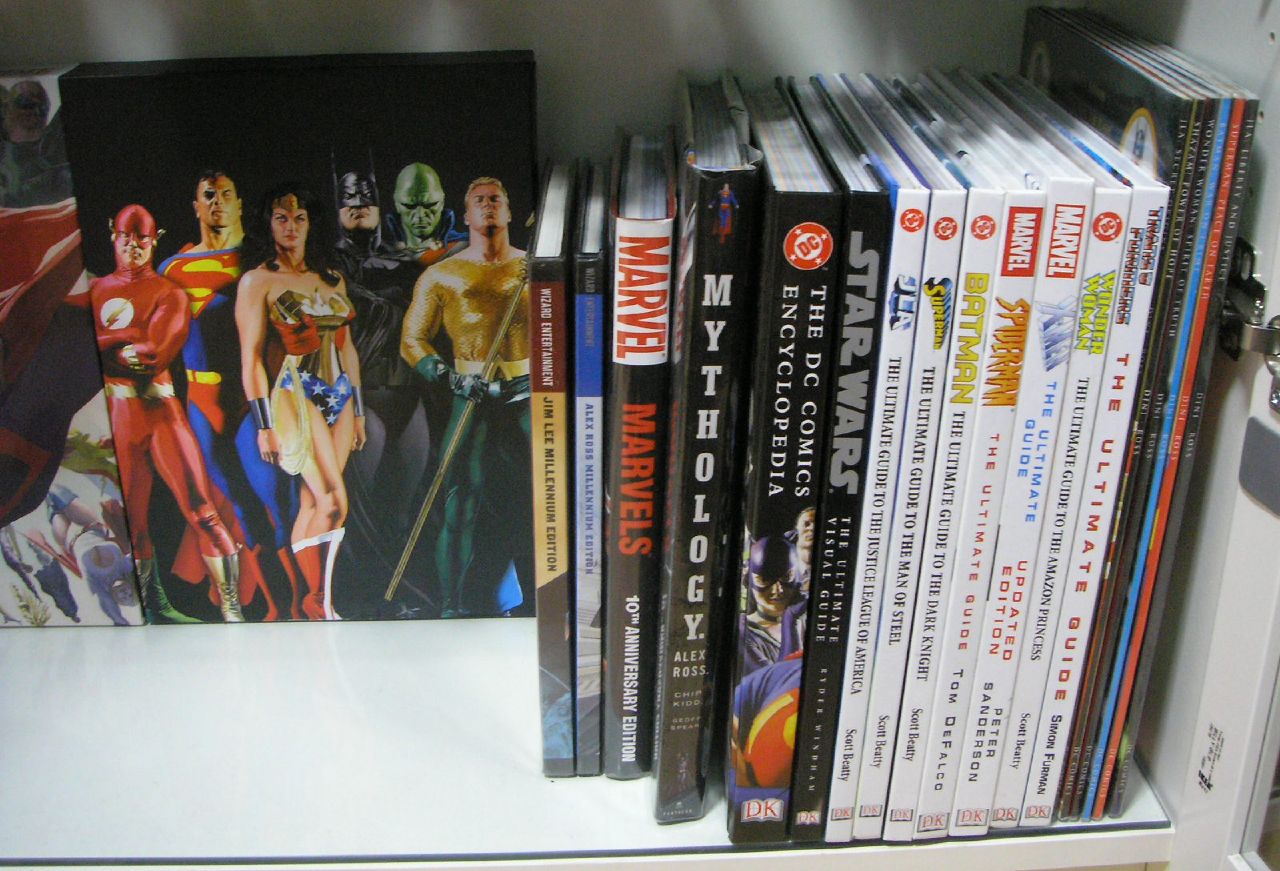This detailed color photograph showcases a pristine white shelf filled with an assortment of books and a vibrant piece of superhero art. On the left side, there's a striking acrylic painting displaying a lineup of iconic superheroes, including Flash Gordon, Superman, Wonder Woman, Batman, a green-headed character, and Thor. Next to this captivating artwork, an array of books is neatly arranged. The first two books have titles too small to decipher, followed by a distinct lineup: "Marvel Marvels," "Mythology," "The DC Comics Encyclopedia," and a "Star Wars" book. Continuing the collection are multiple books with matching covers, each dedicated to famous superheroes such as Superman, Batman, Spider-Man, X-Men, and Wonder Woman, along with "The Ultimate Guide." The final set of six or seven books are noticeably tall and thin, with very tiny titles. All these items are meticulously housed within a clean, white cabinet, representing a well-organized and thematic collection centered around popular superhero and fantasy genres.